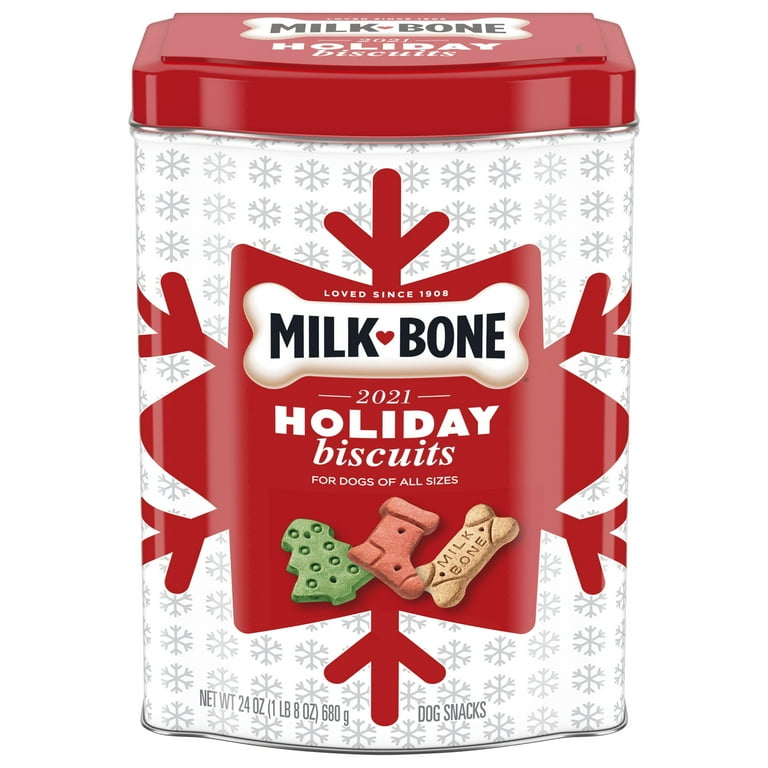This image shows a festive 24-ounce tin container of Milk Bone Holiday Biscuits for dogs of all sizes from 2021. The white tin is adorned with silver snowflakes scattered across a white background and features a prominent red snowflake symbol on the front. The Milk Bone brand logo is prominently displayed, along with the title "2021 Holiday Biscuits for Dogs of All Sizes." The container is rectangular with a red pop-off lid and showcases three holiday-themed dog biscuits: a green Christmas tree, a red stocking, and the classic beige bone-shaped treat embossed with the Milk Bone brand. The label also highlights "Love Since 1908," and provides the weight in both ounces (24 oz.) and grams (680 g).